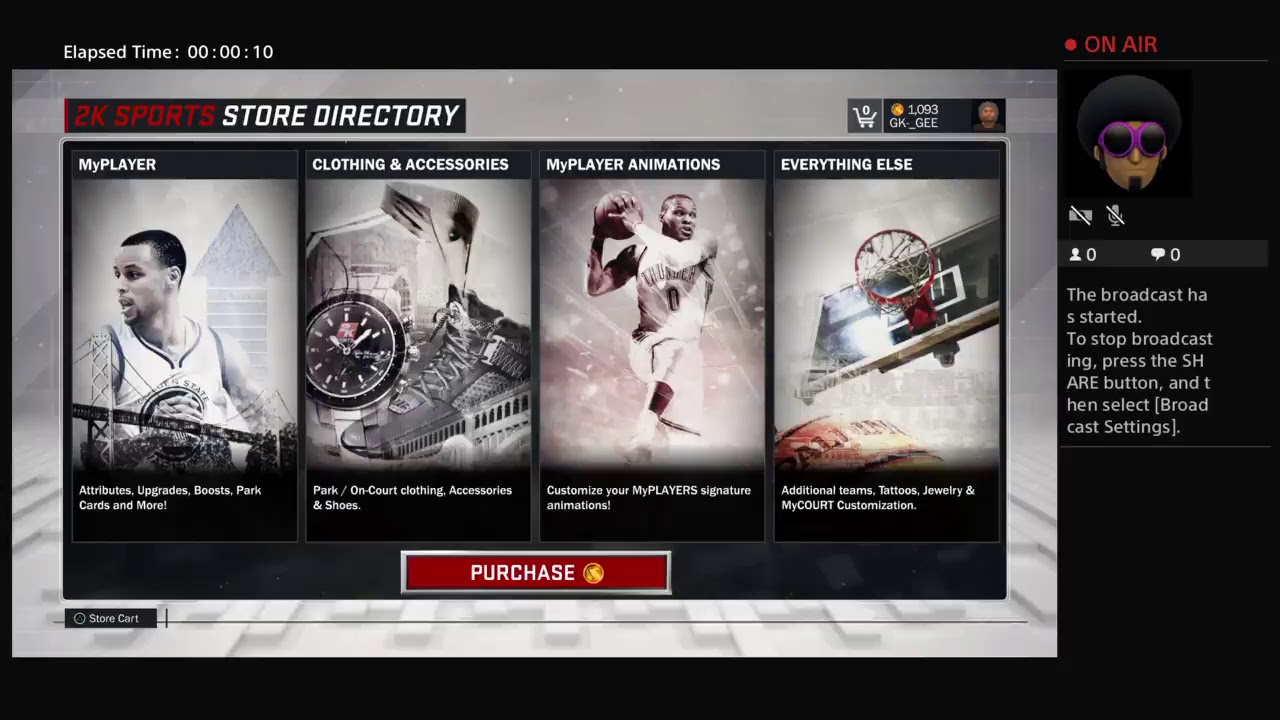**Descriptive Caption:**

Screenshot of an NBA 2K20 or 2K21 video game interface during a live stream broadcast. The background is predominantly black with highlighted text and icons. Centered at the top of the screen in white text is the "Elapsed Time: 00:00:10," indicating the broadcast duration. To the far right, the phrase "ON AIR" is displayed in red next to a red, illuminated record button.

In the main section, there is a profile image of an African-American man sporting a trimmed goatee and pink glasses. Various icons surround the profile pic, including a muted microphone and a crossed-out money symbol. Additionally, a person icon with a "0" next to it (indicating viewers) and a speech bubble icon with a "0" (indicating comments) are displayed. The message, "The broadcast has started. To stop broadcasting, please press the share button and then select broadcast settings," appears prominently.

Below the profile pic, a gray box outlined in black houses several elements: 
- A red "2K SPORTS" logo. 
- A "STORE DIRECTORY" label in white displayed in a smaller, black inset box.
- An avatar icon of the user "GK_dash_GEE" accompanied by a shopping cart with "0" items and "1,093 coins."

The gray box is segmented into four sections, each representing different customizable game options:
1. **My Player**: Featuring a basketball player icon with an up arrow, it offers "Attributes, Upgrades, Boosts, Park Cards, and more."
2. **Clothing and Accessories**: Depicted with icons of sneakers, a watch, and a shirt, detailing "Park/On-Court Clothing, Accessories, and Shoes."
3. **My Player Animations**: Shown with an image of a player performing a jump, it allows users to "Customize My Player Signature Animations."
4. **Everything Else**: Illustrated with a basketball hoop and backboard, it includes "Additional Teams, Tattoos, Jewelry, and My Court Customizations."

At the bottom is a prominent red "PURCHASE" button outlined in black and silver, with a coin icon beside it. Below this button is the "STORE CART" displayed inside a box featuring a circle. The screen's bottom edge has a brick-like pattern along the gray box border, adding texture to the interface design.